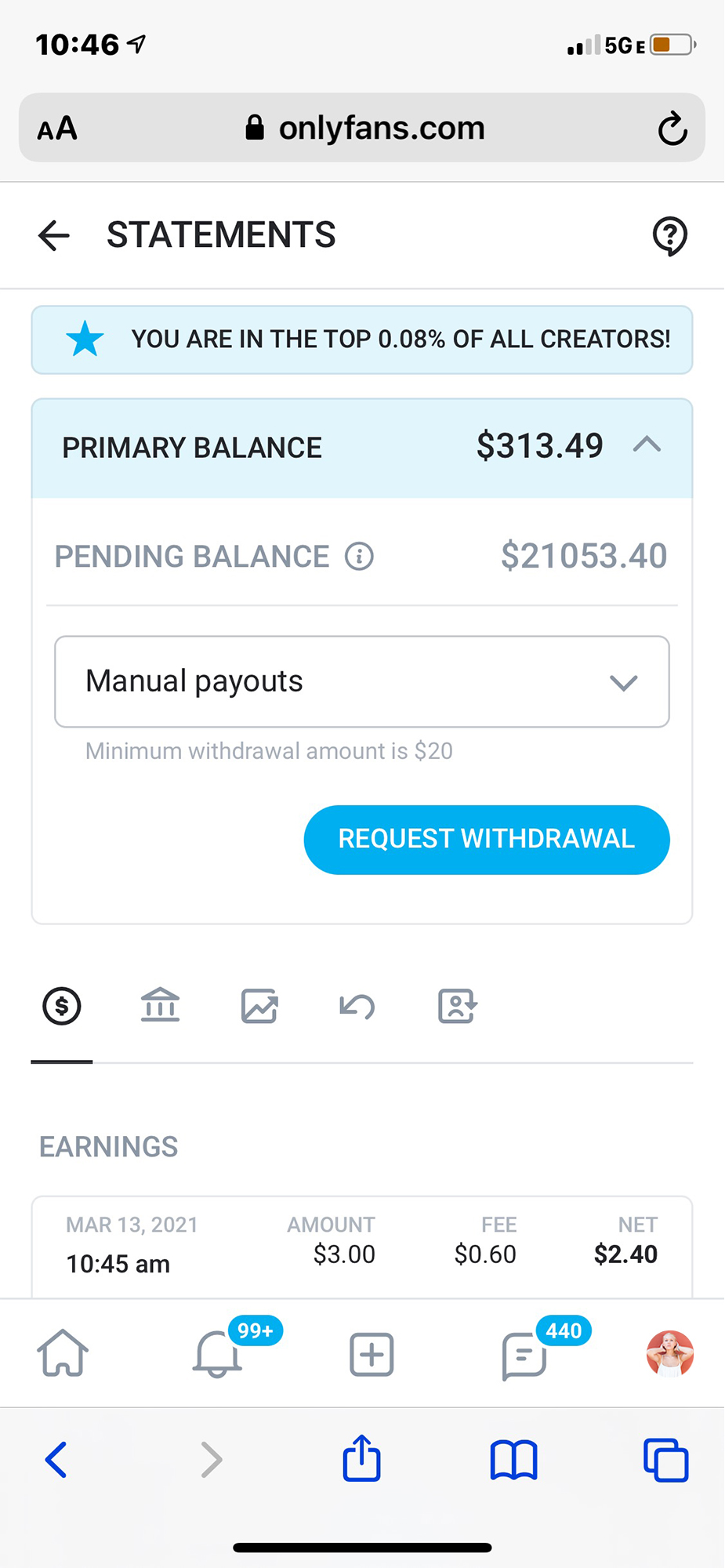This vertical rectangular image, seemingly captured from a cell phone, displays what appears to be a financial dashboard. In the upper left corner, the time is marked as 10:48 in black font, and the upper right corner shows a battery icon at approximately half charge, filled with orange color. Centered in the image is a horizontal oval with "onlyfans.com" in black font, prefaced by a lock icon. Below this, "STATEMENTS" is written with an arrow pointing left.

A horizontal rectangle shaded in blue features a filled star icon on the left, followed by the bold, black, uppercase text: "YOU ARE IN THE TOP 0.08% OF ALL CREATORS!" Directly below, a larger blue-shaded rectangle highlights in bold, uppercase black font: "PRIMARY BALANCE" on the left, with "$313.49" accompanied by an upward arrow on the right.

On a white background beneath, gray uppercase lettering reads: "PENDING BALANCE" followed by an informational "i" in a circle, and "$21053.40" to its right. A horizontal rectangular menu follows, showing "MANUAL PAYOUTS" in black on the left with a down arrow on the right. Below, text advises, "Minimum withdrawal amount is $20." To the right, a turquoise oval button with white, uppercase text says "REQUEST WITHDRAWAL."

Further down, a series of icons are arranged horizontally. The first, a circle containing a dollar sign, is underlined. Other icons follow, and the bottom section notes "EARNINGS" in gray uppercase letters. The date "March 13th, 2021" with a time stamp "10:45 AM" in bold black font is provided. Adjacent columns list "AMOUNT" with "$3," "FEE" with "60¢," and "NET" with "$2.40."